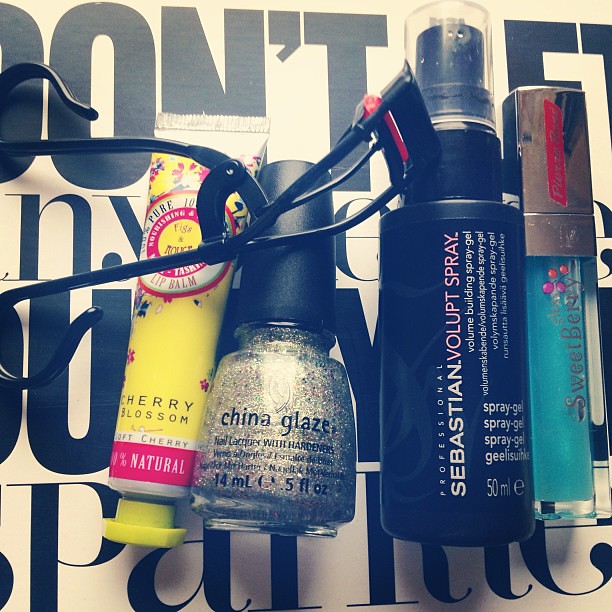This photograph captures an array of personal care and beauty products laid out on top of a white paper with black lettering, though the words are mostly obscured by the items. On the left, there's a black metal eyelash curler with a red rubber piece. Next to it is a tube of 100% natural cherry blossom lip balm, featuring a yellow label with red writing and a matching yellow cap. Moving right, there's a bottle of silver glittery nail polish from the China Glaze brand, adorned with a black cap. Beside that is a black bottle of Sebastian Volupt Spray with a clear cap, labeled in white as a volume-building spray gel containing 50 milliliters. On the far right lies a long, slender bottle of light blue lip gloss, labeled "Sweetberry," and topped with a silver metallic cap. All items are carefully arranged on the white paper, partially covering the bold black text beneath them.